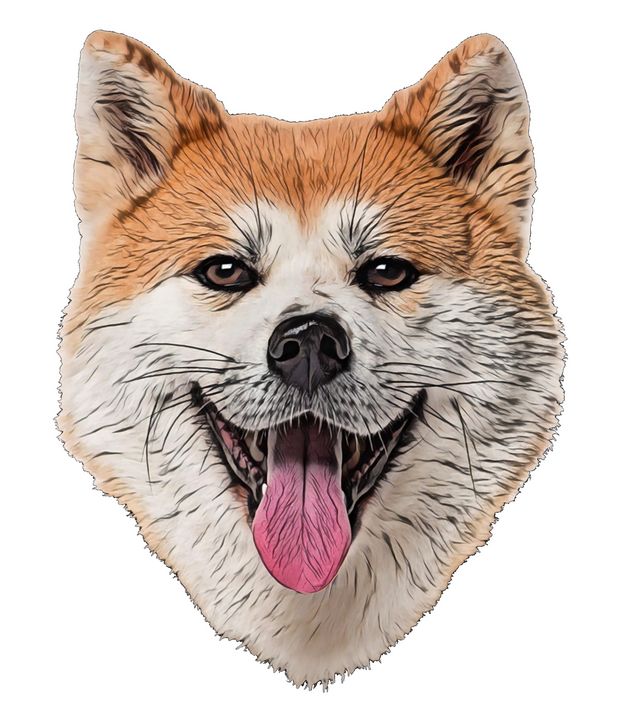This is an intricately detailed color illustration of a dog's head, prominently featuring attributes of breeds like the Shiba Inu, collie, or husky. Set against a stark white background, the dog's visage is captured with a pronounced realism while maintaining a drawn graphic quality. Its fur is a combination of rich, reddish-brown tones above the eyes and on the ears, blending seamlessly into a white-beige hue around the lower face and cheeks, giving it a mane-like appearance streaked with black lines.

The ears are short, triangular, and stand attentively upright, with light tan and a touch of black shading inside. The dog's eyes are a compelling brown or amber, exuding friendliness and warmth, with reflective highlights that add to their lifelike quality. Above the eyes, distinct black eyebrow hairs protrude, complemented by black whiskers near a damp-looking black nose.

The dog's mouth is open in a cheerful expression, revealing a pink tongue detailed with fine lines and some white lower teeth on either side of the tongue. The overall texture of the fur is accentuated by black lines, emphasizing the illustration's meticulous attention to detail.